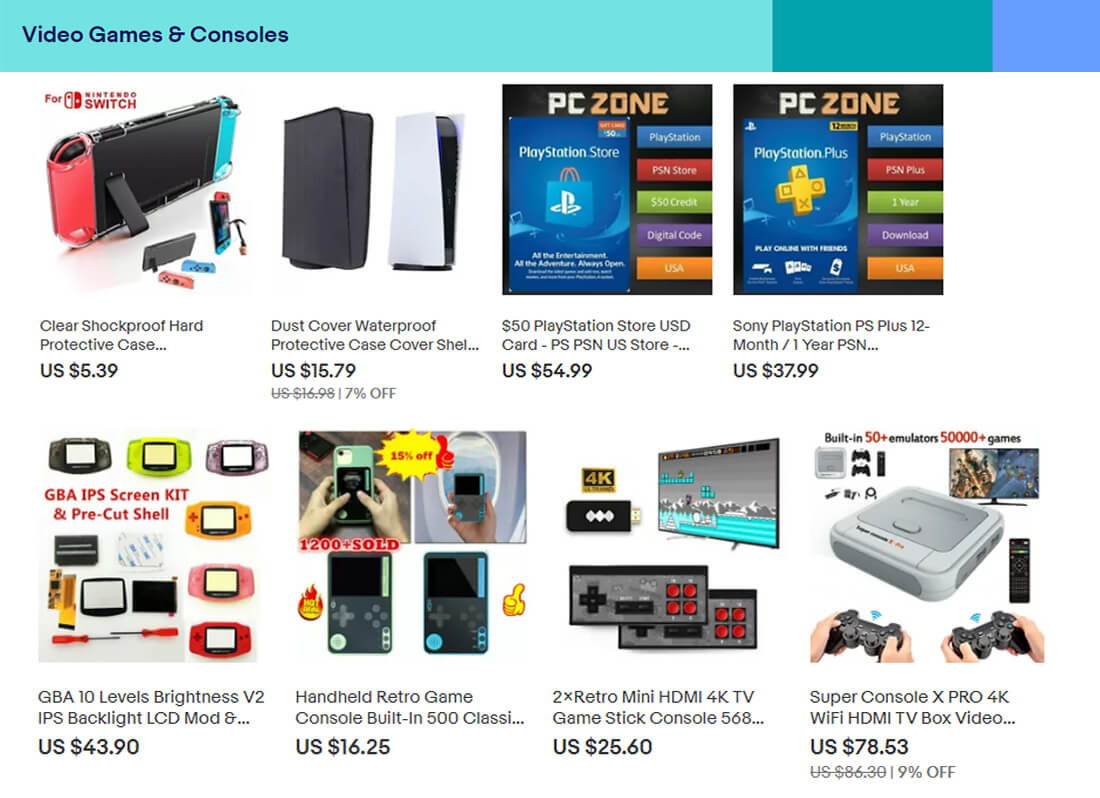This is a low-resolution, artifact-laden, cropped image of an older store page, indicative of a screenshot shared multiple times. The page has a dated design with a banner at the top composed of three blocky shades of blue, primarily a teal hue stretching across three-quarters of the image, accompanied by two darker shades clustered at the end. Black text on the banner reads "Video Games and Consoles."

The main section features a grid layout on a white background, organized in a 4x2 format, displaying various video game-related items and equipment. The items are as follows:

1. A Nintendo Switch enclosed in a clear, shockproof, hard protective case, priced at $539.
2. A PlayStation 5 console.
3. PlayStation Store and PlayStation Plus gift cards.
4. A Game Boy Advance IPS screen kit displaying a lit LCD screen, depicted with multiple Game Boys.
5. A retro game console resembling a budget Game Boy.
6. Two retro mini HDMI 4K TV game stick consoles.
7. Another inexpensive console that mimics the aesthetic of an old Super Famicom but is paired with PlayStation-style controllers, named the Super Console X.

The visual quality of the page makes it difficult to discern finer details, reinforcing the impression of it being an aged or often-shared screenshot.